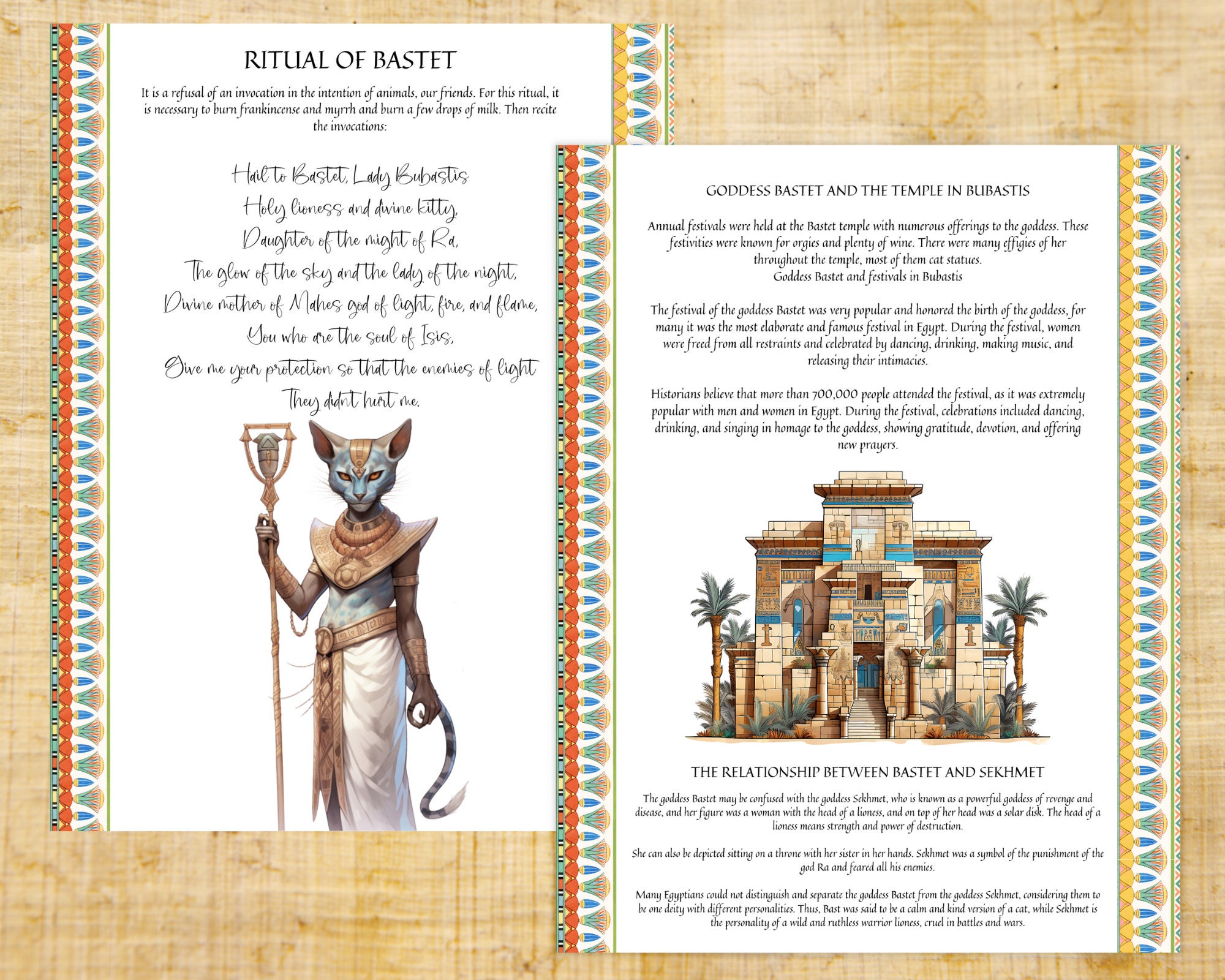The image consists of two illustrated posters, each highlighting aspects of the Egyptian goddess Bastet. The left poster, titled "A Ritual of Bastet," depicts Bastet as a human-shaped cat dressed in traditional Egyptian royalty attire, including a dress with a gold belt and a necklace. She holds a large staff in her right hand. The text under the title is difficult to read but includes phrases like "Hail to Bastet, Lady Bastet, holy goddess," and mentions her divine relationship as the "daughter of the glow of the sky and the lady of the night." The intricate handwriting and small font size make the detailed text largely illegible.

The right poster illustrates an Egyptian temple with two pillars, a tower, and gabled roofs, flanked by palm trees. This image is accompanied by the title "Goddess Bastet and the Temple in Bubastis." The text below touches on the annual festivals held at the temple, celebrating the birth of Bastet, and notes the festival's popularity among Egyptians, with attendance reaching over 100,000 people. Additionally, the poster discusses the relationship between Bastet and another goddess, Sekhmet. Both posters are set against a brown paper background, with white paper featuring red and green borders framing the illustrations and text.